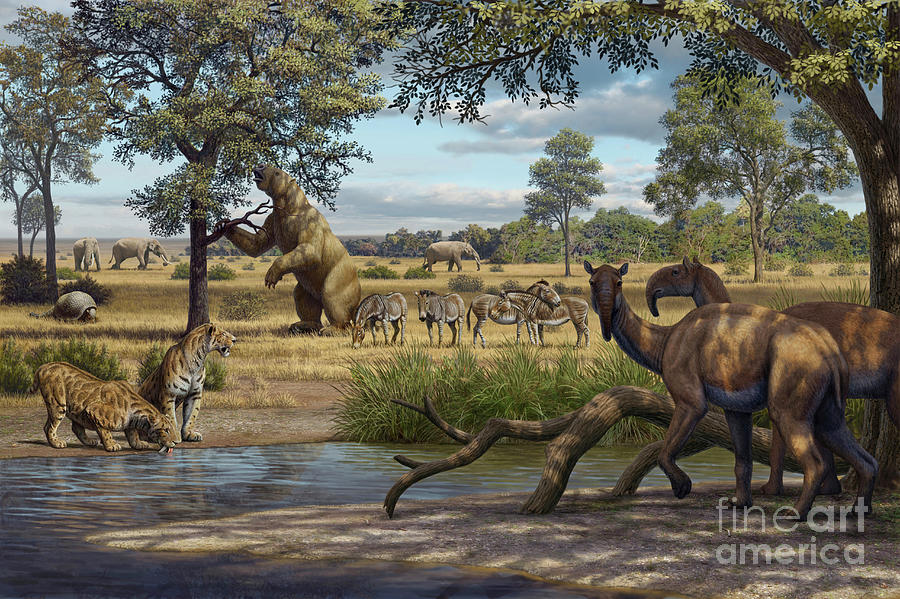The image is a detailed, vibrant painting of an African savanna teeming with a diverse range of wildlife, including both modern and prehistoric-looking animals. The landscape is set in the morning under a clear sky, with numerous trees dotting the background and foreground. In the center of the composition are four zebras with a dusty brownish hue, grazing on yellow grass. A colossal bear stands prominently among the zebras. 

To the left, near a pond, two tigers drink water, and nearby, a large tortoise or a similarly shelled creature is seen. Farther to the left, there are three elephants scattered across the scene – one in the back, one toward the middle, and another further in the distance. On the right side of the painting, peculiar large creatures resembling anteaters walk near another tree. Additionally, animals resembling a camel without humps or mules are visible, adding to the eclectic mix of wildlife. 

The bottom right corner of the painting features a watermark reading "Fine Art America," affirming the source of this captivating artwork.